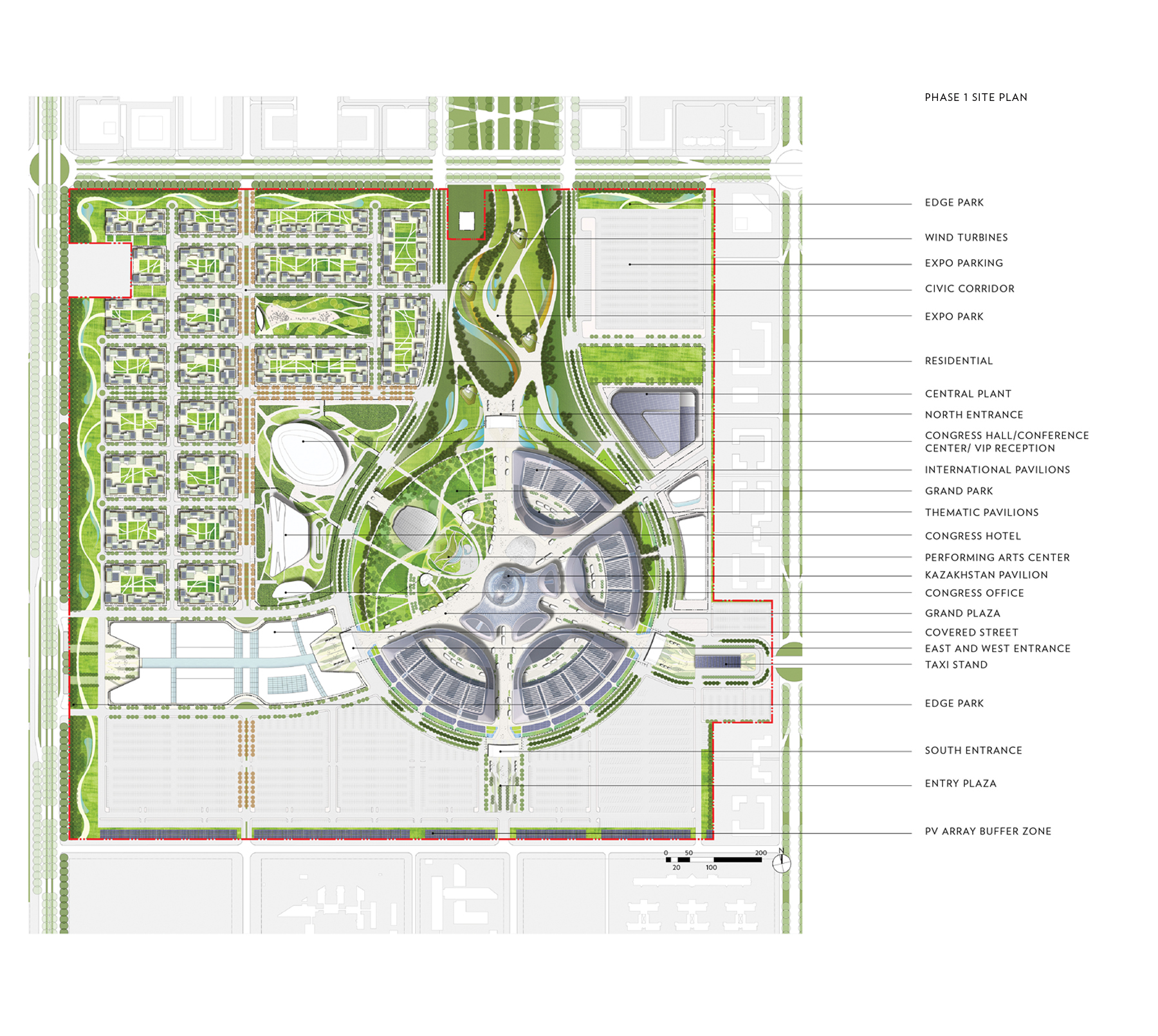The image depicts a detailed and intricately labeled Phase 1 Site Plan for a planned development, potentially located in Asia, as it includes a Kazakhstan Pavilion. The schematic, predominantly green and gray, features various parts of the site meticulously labeled on the right-hand side along with a measurement bar and a compass at the bottom center. The site plan outlines numerous zones and facilities including Edge Park, Wind Turbines, Expo Parking, Civic Corridor, Expo Park, Residential Central Plant, North Entrance, Congress Hall, Congress Center, VIP Reception, International Pavilions, Grand Park, Thematic Pavilions, Congress Hotel, Performing Arts Center, Kazakhstan Pavilion, Congress Office, Grand Plaza, Covered Street, East and West Entrance, Taxi Stand, South Entrance, and PV Array Buffer Zone. The central design highlights the interconnected layout and forthcoming attractions, showing the strategic plan for this expansive outdoor plaza and its various amenities.